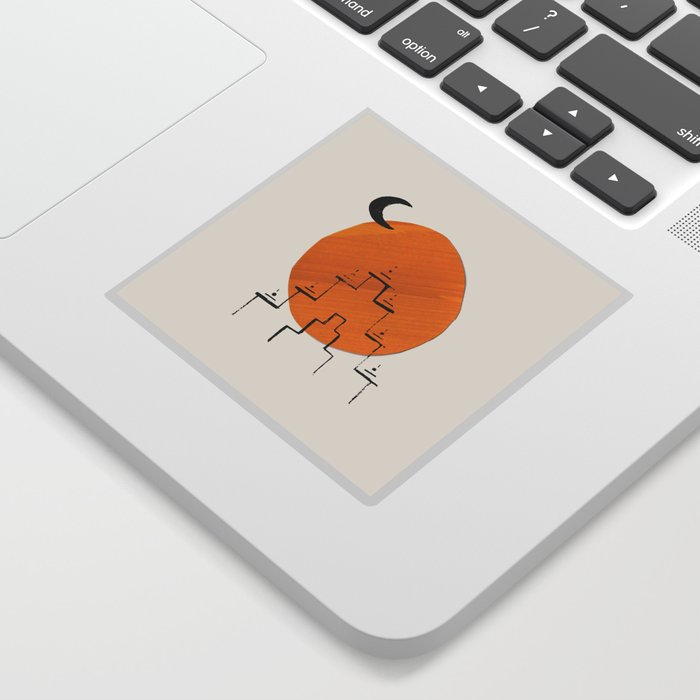The image portrays the bottom right corner of a silver MacBook laptop keyboard, positioned on a plain white surface. A small square sticker is affixed next to the trackpad, on the right side. The sticker features a light beige background with a prominent orange circle in the center, representing the sun. To the top left of the sun, a small black crescent moon is sketched. Below the sun, there is a drawing of a tiered temple-like structure. The visible keyboard keys include the arrows, shift, option, and question mark keys. The laptop's speaker area can also be seen.